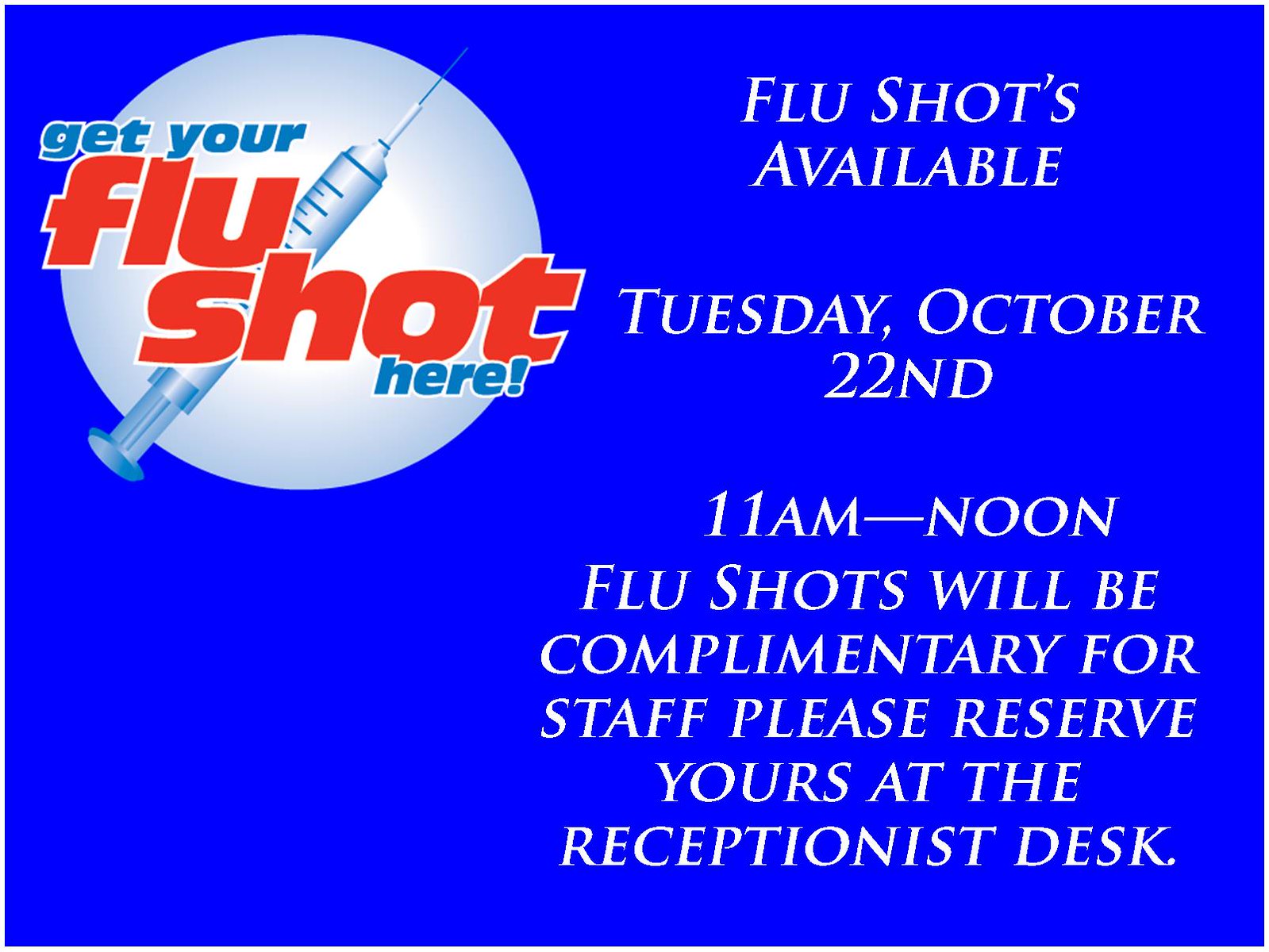This digital advertisement features a predominantly blue rectangular layout, designed to promote flu shots. In the top left corner, there's a grayish-white circle resembling a moon or a ball, overlaid by a clipart-style syringe. The prominent text on this circle reads, "Get your flu shot here," with "get your" and "here" in light blue with white outlines, and "flu shot" in bold red with white outlines. 

The main body of the ad, set against the royal blue background, contains white text that details the event: 

"Flu shots available Tuesday, October 22nd, 11 a.m. to noon. Flu shots will be complimentary for staff. Please reserve yours at the reception desk."

The design is simple yet effective, featuring clean and easy-to-read text. Though there is an unnecessary apostrophe in "flu shots," the overall message remains clear and informative. The ad is likely intended for an office or break room bulletin board, encouraging staff to take advantage of the complimentary flu shots offered.